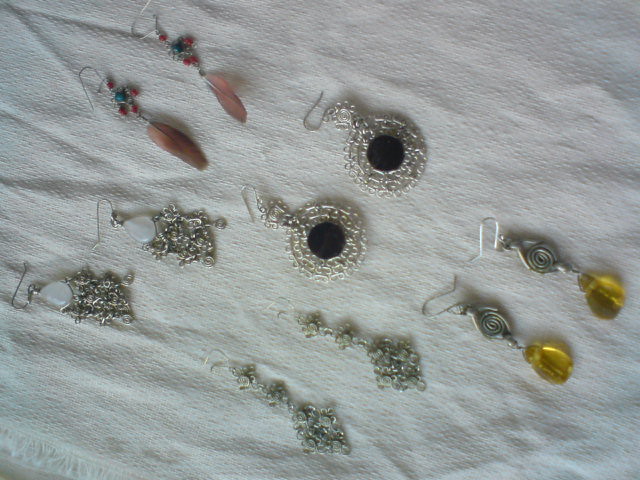This photograph captures an array of dangle earrings meticulously spread out on a white cloth surface that bears the texture and worn look of a slightly rough dish towel or perhaps a scarf, complete with a frayed edge in the lower left corner. Each earring is designed for pierced ears and showcases a variety of intricate styles. In the upper left corner, there are earrings featuring red feathers hanging down from a centerpiece adorned with small red and blue jewels. Adjacent to these, a silver pair with a mass of delicate swirls culminate in a white pearl. Further right, earrings with silver, triangle-like frames offer a unique textured design. Below these, a pair of silver earrings with a circular form enclose a striking black center. Another pair, evocative of chains, boasts diamond shapes attached to green-tinted silver circles. To the far right, there are silver earrings with an intricate swirl design accented by yellow stone droplets, exuding a rugged charm. The assortment captures the diversity and beauty of earring designs, from feather-adorned to gem-encrusted creations.